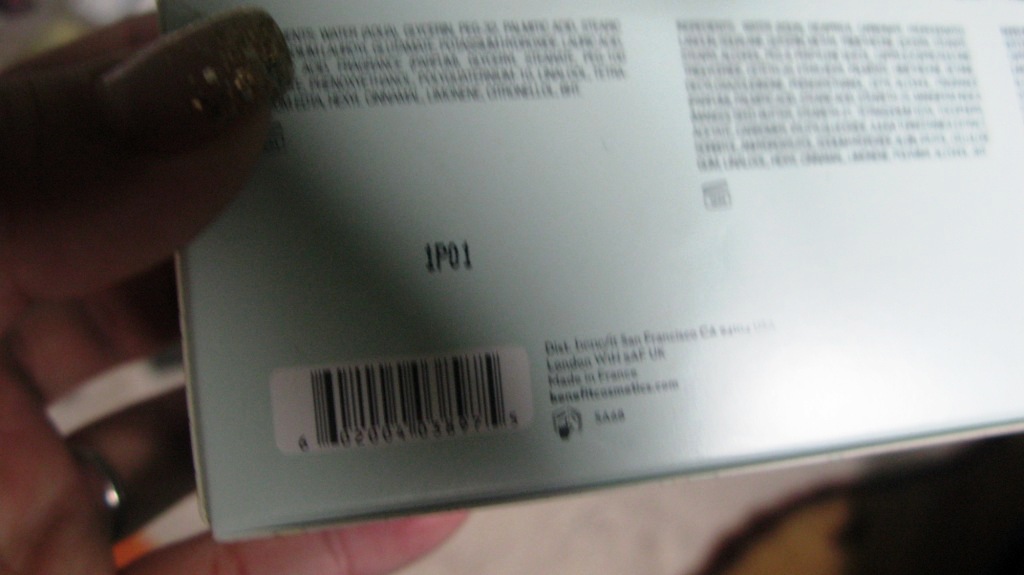This image is a close-up, color photograph depicting a person's left hand holding the lower left-hand corner of a box. The photo is notably blurry and out of focus, making the details of the box and its text rather indiscernible. The hand, with a medium complexion, wears a wedding ring on the fourth finger and features a manicured thumbnail with dark polish and gold sparkles. The box appears to be rectangular and is held in a portrait orientation, showcasing a white barcode at the bottom left corner with the code IP01 stamped above it. Partially legible text includes "DIST. BENEFIT SAN FRANCISCO. LONDON. MADE IN FRANCE. BENEFITCOSMETICS.COM," hinting that the product may be from Benefit Cosmetics. The background consists of a white surface with a dark and light brown curve in the lower right-hand corner.